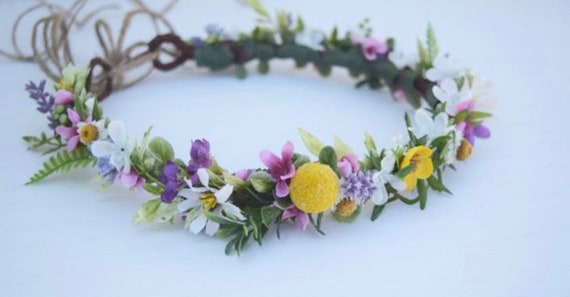This photograph features a vibrant flower crown resting against a backdrop that appears pale blue due to shading effects, despite the white background. The flower crown is crafted as a circlet designed to sit atop the head or around the forehead. It includes adjustable sizing with two rings at the back linked by a string. The florist's tape securing the arrangement is dark green, blending seamlessly with the natural elements. The crown showcases an array of fern leaves, fern flowers, and assorted greenery, interspersed with an exuberant mix of white, purple, pink, and yellow flowers of various species. This delightful combination exudes a joyful, springtime ambiance.